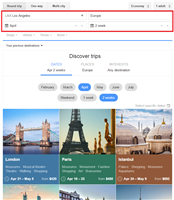This screenshot depicts a highly blurry travel website page, making the exact details challenging to discern. The image quality is very poor, contributing to the difficulty in reading most of the text. It features a predominantly white background.

At the very top of the page, there is a search box outlined in red, likely indicating "from" and "to" fields for booking flights. The departure appears to be from "LAX" in Los Angeles, although the destination is unreadable.

Centered below the search box is the phrase "Discover Trips." On the left, the section labeled "Dates" is indecipherable due to blurriness. In the middle, there's a section labeled "Places," and on the right, it appears to be labeled "Destination."

The page includes several gray oval shapes with abbreviated or full month names inside them. The months listed include February, March, April (highlighted in blue), May, June, and July. Below this row, there is another set of options with labels for trip duration: "Weekend," "One Week," and "Two Weeks," with "Two Weeks" highlighted in blue.

The bottom section of the image displays three photographs. The left photo is labeled "London" and shows the London Bridge. The middle photo is labeled "Paris" and features the Eiffel Tower. The right photo is unclear, but it depicts two large dome structures. The label for the rightmost photo is unreadable.